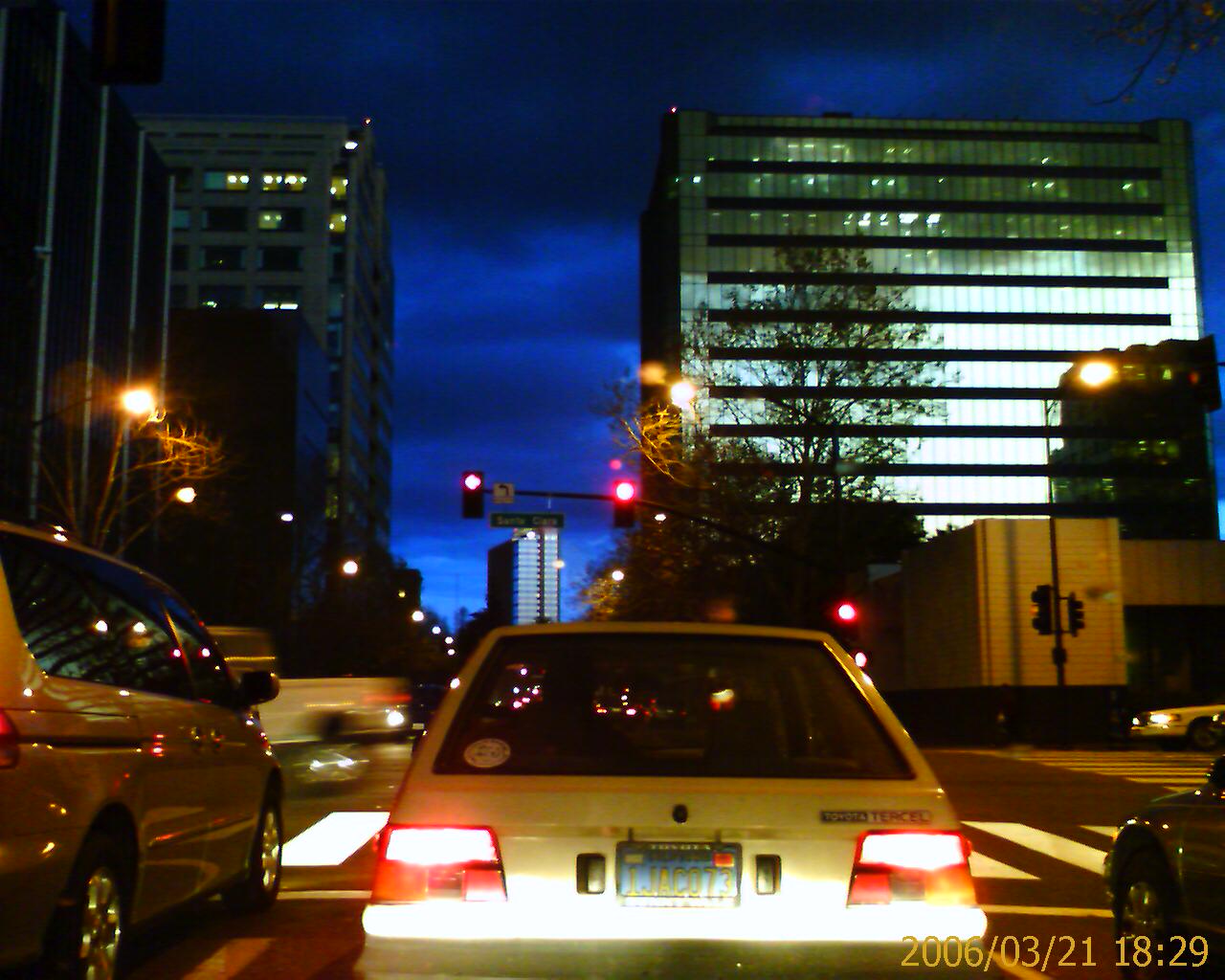The image depicts a close-up night scene taken from the windshield of a car stopped at a red light. Central to the image is a small white station wagon-like car, with its bright brake lights glowing, positioned in the bottom center. To its left, part of a gray minivan is visible, while the bottom right corner reveals a portion of another small, dark-colored vehicle. A yellow timestamp at the bottom right reads 2006-03-21-18-29. Above the car in the mid-background, two skyscrapers flank either side of the street, with another, more distant one centered between them. Street lamps light the road, while overhead, dark clouds accentuate a twilight sky in varying shades of deep blue. A traffic light pole spans the road, displaying two red lights and a crosswalk indicator, mirroring the red brake lights from the cars below. A white sign with a black arrow pointing left hangs beneath the traffic lights, completing the detailed scene.